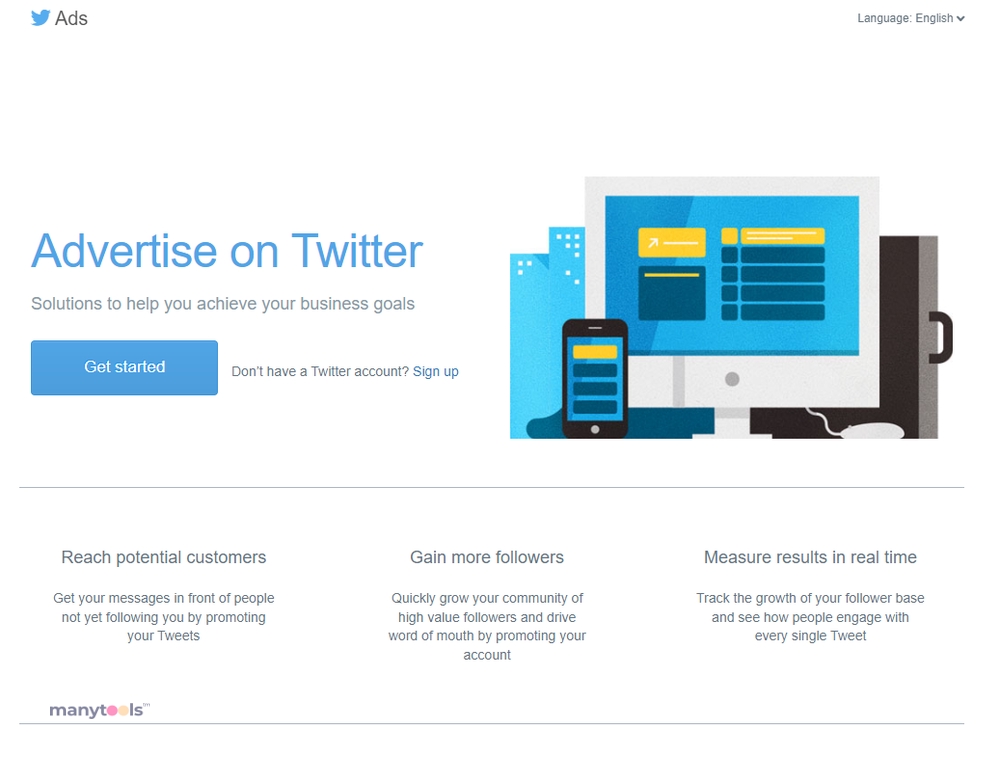This detailed screenshot from Twitter, featuring a classic white background, highlights an advertisement for the platform’s promotional services. At the top left corner, the recognizable Twitter icon is displayed next to the word "ads." The main heading on the page, shown in prominent blue text, reads "Advertise on Twitter." Just beneath it, a smaller black text provides a succinct description: "Solutions to achieve your business goals." 

Below this informative text, a blue "Get Started" button is prominently positioned alongside a "Sign Up" link, inviting users to begin their advertising journey. On the right side of the screenshot, a computer-generated graphic illustrates a silver-cased computer monitor perched on a stand, alongside a black-cased mobile phone. Both devices display a web page with a cohesive blue and orange color scheme, featuring charts on the computer screen's blue background and a similar blue screen on the mobile phone.

Adding a touch of professionalism, a black briefcase is positioned behind the computer monitor. The middle section of the web page is divided into three distinct columns: "Reach potential customers," "Gain more followers," and "Measure results in real time," each summarizing key benefits of advertising on Twitter.

Finally, the bottom left corner of the screenshot includes gray text that reads "many tools," with the "O"s in "tools" creatively highlighted in pink and peach. This comprehensive snapshot effectively conveys the various features and benefits of utilizing Twitter for business advertising.